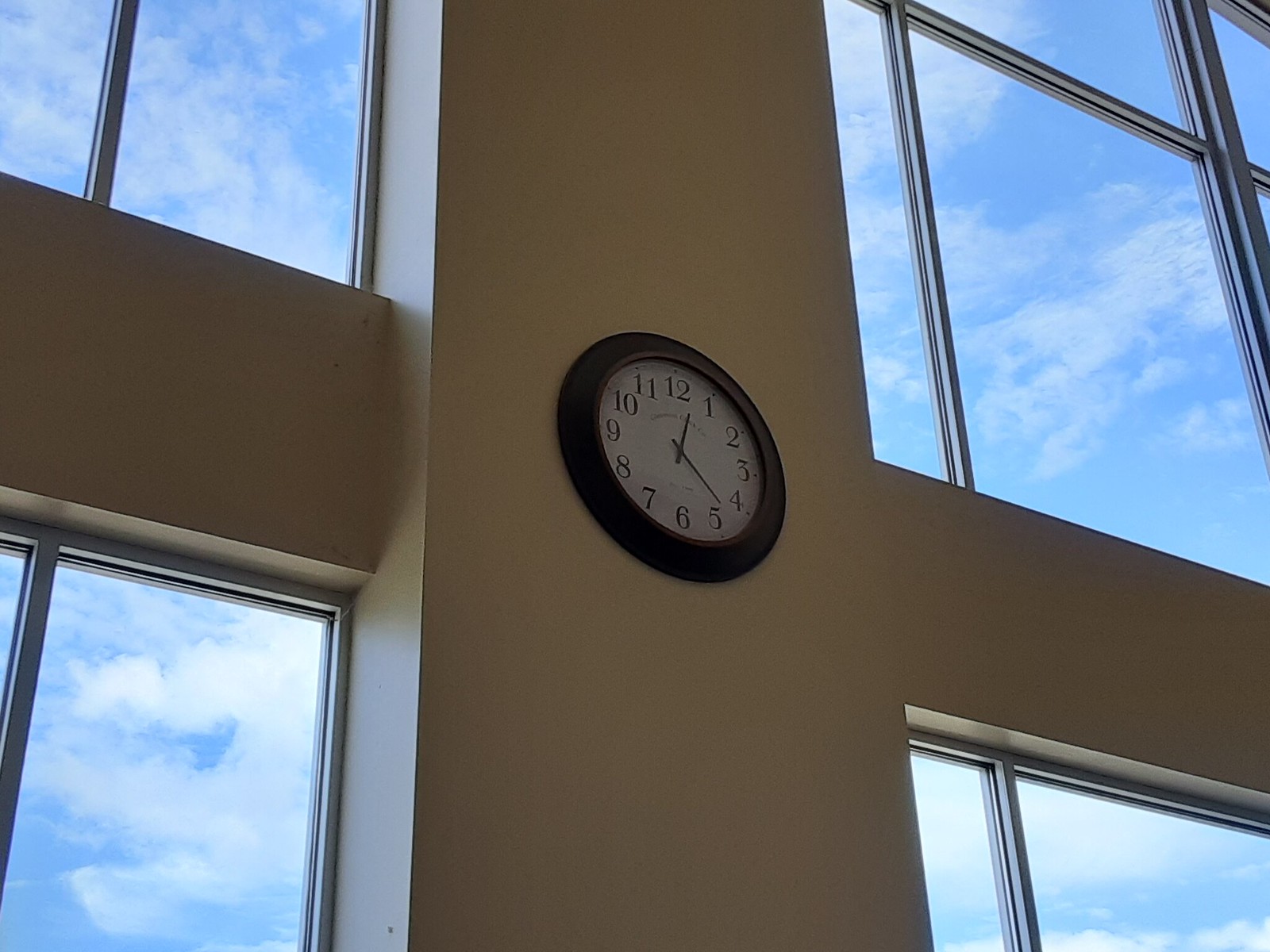A white, circular clock with a black border is mounted on a wall that intersects in a cross shape, created by one vertical beam meeting a horizontal beam. The clock, featuring minimalist straight lines as its hour and minute hands, shows a time of approximately 12:23, with the shorter hand positioned between the 12 and 1, and the longer hand between the 4 and 5. Surrounding the clock, the wall is flanked by four large windows located at the top left, bottom left, top right, and bottom right corners. These windows have sleek, grayish-black frames divided into a grid-like pattern, offering a view of a blue sky scattered with small clouds.